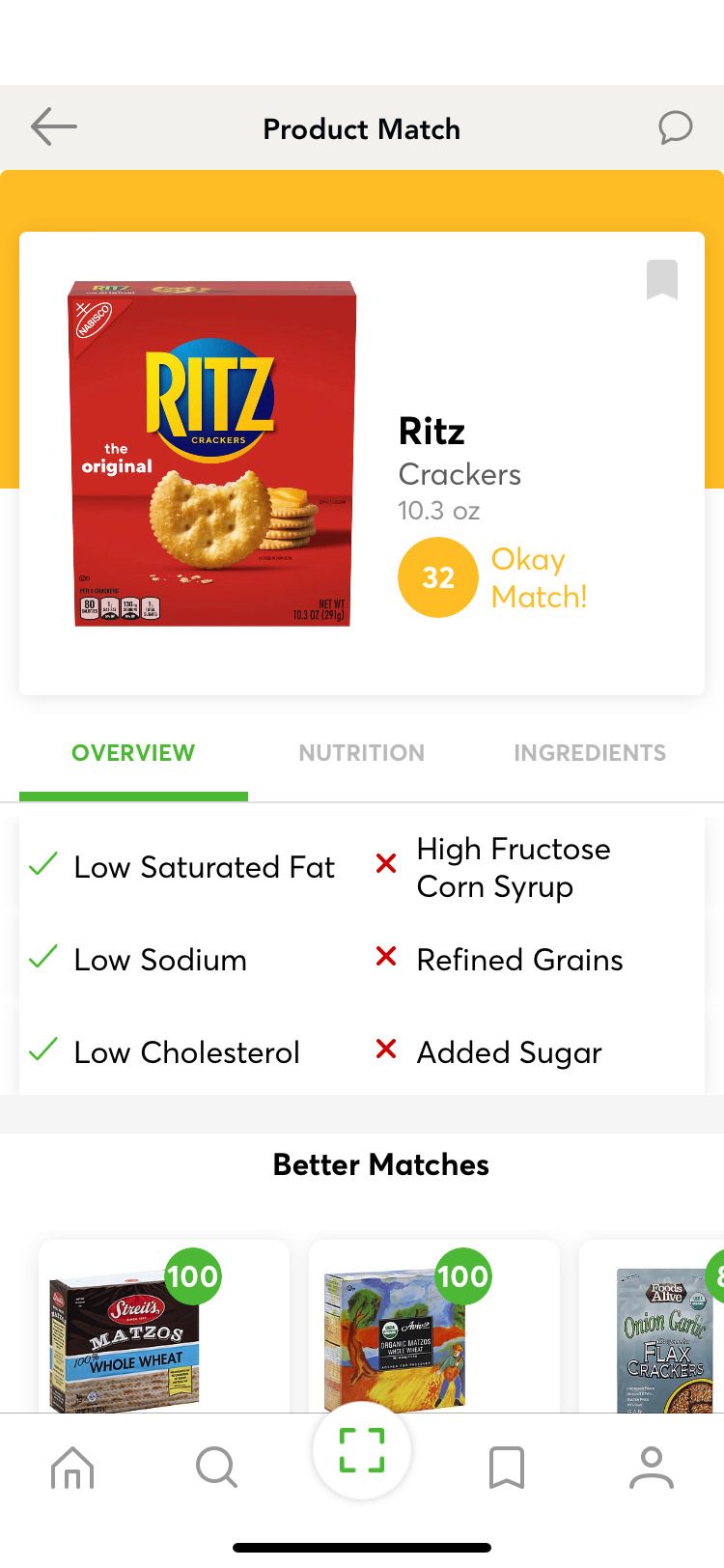The image displays a website called "Product Match," prominently featuring a box of Ritz Crackers at the top. The Ritz Crackers box is red with "The Original" written on it and features the Nabisco brand name in the upper left corner. The box displays an image of the crackers, with one cracker standing on its edge and a bite taken out of it. Behind this cracker is a stack of additional crackers. 

The title "Ritz Crackers 10.3 ounces" is displayed near the top. Next to it, there's an orange circle with the number 32 inside. Above the Ritz Crackers image, there is an orange border, and below it, the word "Overview" is shown in green and underlined. To the right of "Overview," the words "Nutrition" and "Ingredients" appear in gray.

Below the "Overview" section, nutritional summaries are provided: "Low Saturated Fat," "Low Sodium," and "Low Cholesterol" are displayed with check marks, while "High Fructose Corn Syrup," "Refined Grains," and "Added Sugar" have red Xs next to them.

Under the nutritional summaries, the "Best Matches" section is displayed, showing comparable products. It includes a box of whole wheat matzos, marked with a green circle containing the number 100. There is also another product, with a tan-colored box and another green circle with the number 100, though the image is small and hard to distinguish. Lastly, an item with what appears to be Asian writing is shown, but the green circle is cut off, making it unreadable.